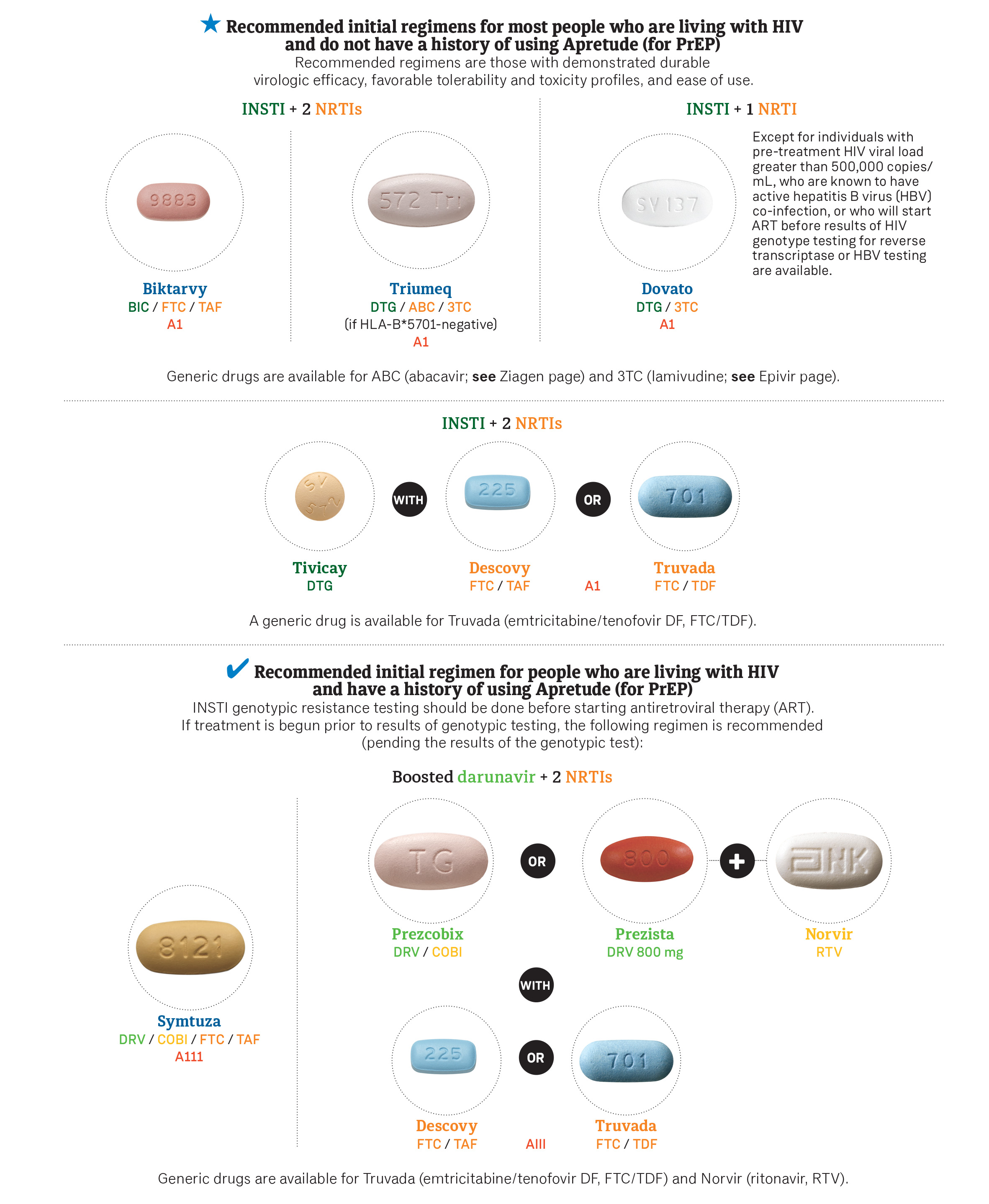This image showcases various antiretroviral medications for people living with HIV. At the top center, a statement reads: "Recommended initial regimens for most people living with HIV who do not have a history of using Apretude (for PrEP)." Below this, in a lighter font, it notes: "Recommended regimens are those with demonstrated durable virologic efficacy, favorable tolerability and toxicity profiles, and ease of use." 

The image features three primary sections, each highlighting a specific pill. 

1. The first square displays the medication BIKTARVY, an oval, pinkish pill with the imprint "9883."
2. The second square shows TRIUMEQ, represented by a white pill.
3. The third square presents DOVATO, a lighter white pill.

Below these three sections are two additional sections, each featuring a pill accompanied by a detailed description.